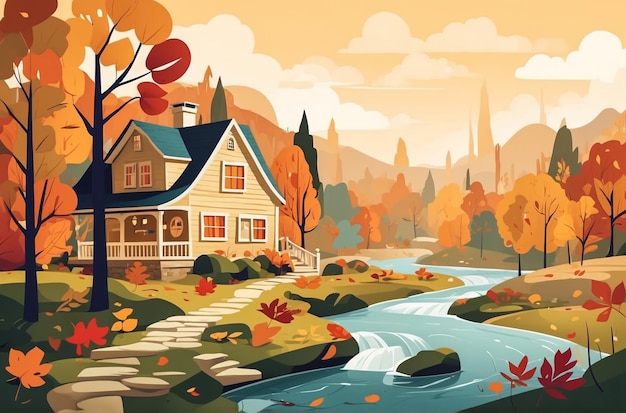In this autumnal, cartoon-style painting, a cozy, tan cottage with a blue roof sits in the left-hand corner of the image, surrounded by vibrant fall foliage. The house features a quaint covered porch and multiple windows, including a circular one adding unique charm. A cobblestone path with stepping stones and stairs, complete with a railing, leads from a rushing light blue stream up to the cottage's front door. This stream winds from the foreground through the middle of the scene, dotted with floating orange leaves. Tall trees with a mix of orange, brown, and reddish leaves frame the house, their leaves carpeting the ground below. Hills and more autumn-colored trees populate the background, enhancing the painting's tranquil, rustic atmosphere. The limited, almost posterized color palette emphasizes the warm and cozy feeling of this idyllic autumn day.